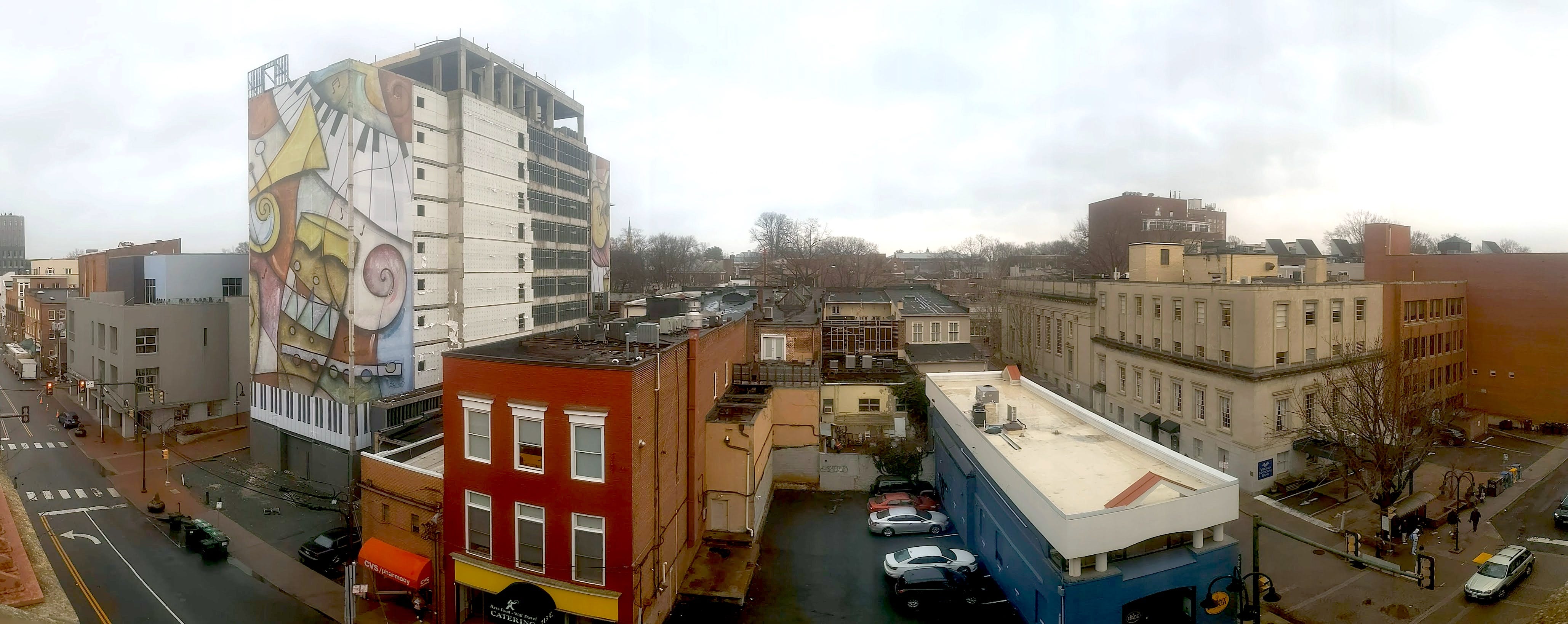This panoramic view captures the urban landscape of Harlem, Manhattan, New York City, on an overcast day. Prominently featured is a large, colorful building adorned with a mural depicting musical themes, including pianos, drums, and keyboards. This mural embellishes both the front and sections of the building, integrating piano keys along the sides. This standout structure, approximately 10 stories high, is situated along Frederick Douglass Boulevard, surrounded by a variety of buildings—some gray, some red, and some blue—ranging from two to three stories high. The scene also includes a street with parked cars, a small parking garage, and an alleyway, contributing to the bustling atmosphere of this iconic urban neighborhood.